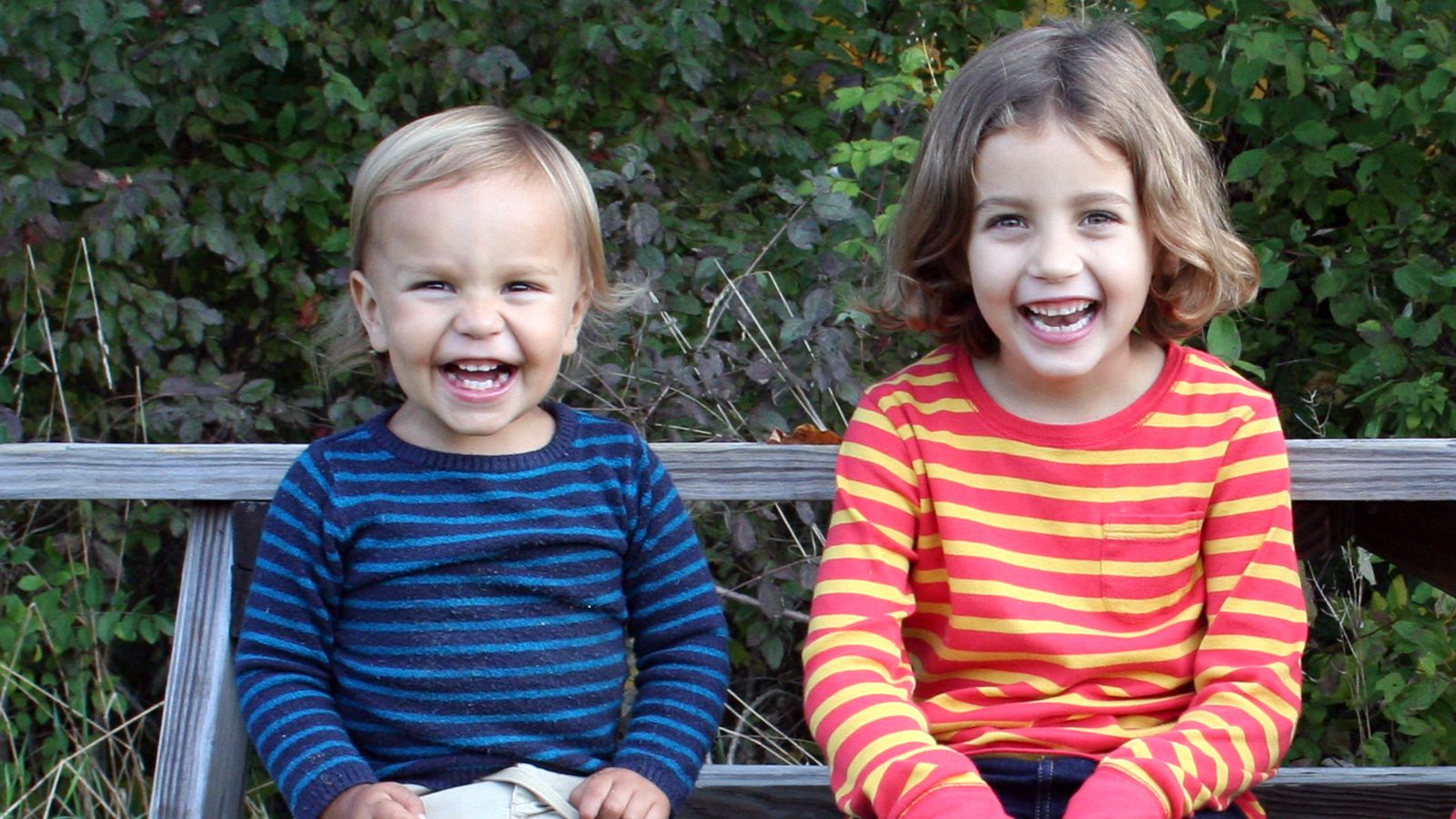In the photograph, two young girls, likely sisters, are seated on a weathered light brown wooden picnic table, with their upper bodies visible. Their joyous expressions feature wide, open-mouth smiles that highlight their familial resemblance. The girl on the left, the younger sibling, has medium-length blonde hair parted on the side and wears a light blue and dark blue striped sweater. The older girl on the right has shoulder-length, slightly darker brown hair and dons a pink and yellow striped shirt with a button or a pocket on the front. Surrounding them is a background of varying foliage, with darker, muted leaves on the left and brighter, more vibrant leaves on the right. The setting also includes a dark grey, wood-like fence structure extending behind them, contributing to a cozy outdoor atmosphere.